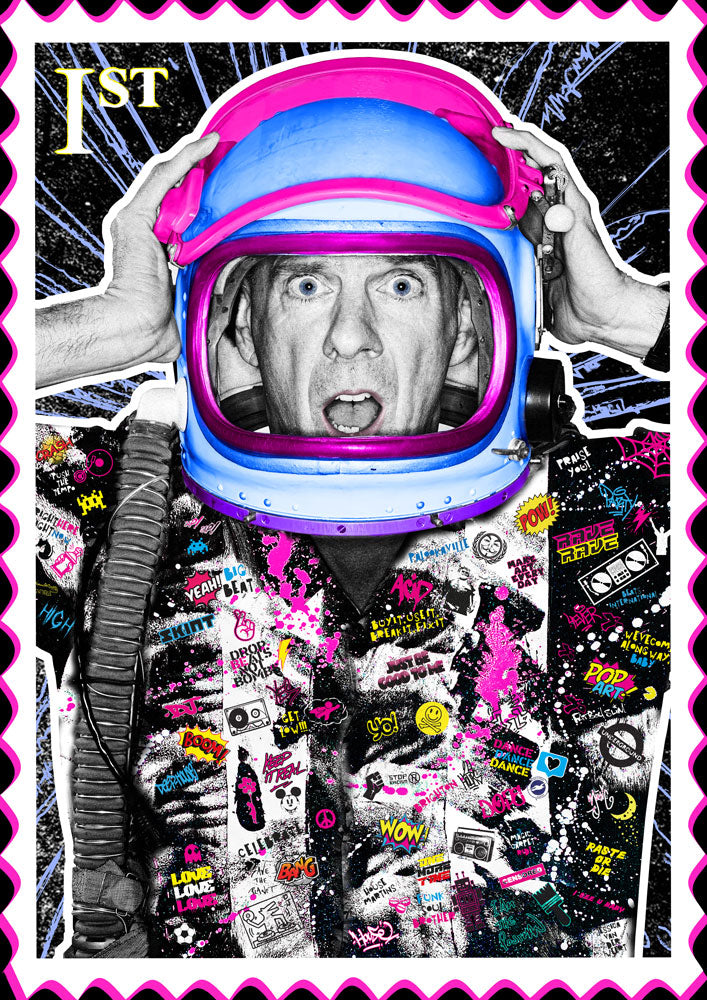This vibrant digital artwork resembles a stamp, featuring a man with a shocked expression, eyes wide and mouth agape. At the top left corner of the stamp, there is a "1ST" designation. The man wears an astronaut helmet, with a flipped-up visor, painted in striking neon pink and blue hues. His face and hands are rendered in black and white, enhancing the contrast against the colorful helmet. He holds his head with both hands, further emphasizing his surprised demeanor. 

The man's torso is adorned in an astronaut suit covered with an eclectic mix of graphic street art and graffiti-style stickers. These vivid, comic book-esque stickers feature words and phrases such as "pow," "yeah," "love, love, love," "drop," "no bomb," "wow," "dance, dance, dance," "yo," "rave," and "raste or die." The suit also displays spider webs, paint splatters, peace signs, and even a Pac-Man image, all executed in neon colors like pink, yellow, blue, and purple. Additionally, a tube, possibly an air supply, hangs from the right side of his helmet and travels down his front. The artwork is framed with a design of scallops, black with purple edging, enhancing its detailed, pop art aesthetic.